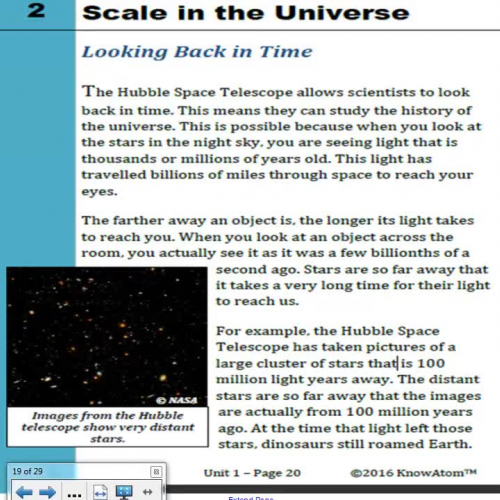This image captures a published article from a textbook, specifically displaying Unit One on page 20. The article, titled "Scale and the Universe: Looking Back in Time," discusses themes related to the Hubble Space Telescope. A noticeable copyright mark, attributed to KnowAtom (spelled K-N-O-W-A-T-O-M), is present in the lower right-hand corner, dated 2016. The bottom left corner of the image features a striking photograph of the cosmos, showcasing a star-filled, black expanse of outer space. The layout and content suggest that this publication is likely an educational piece aimed at providing in-depth knowledge about the universe and the instruments used to explore it.